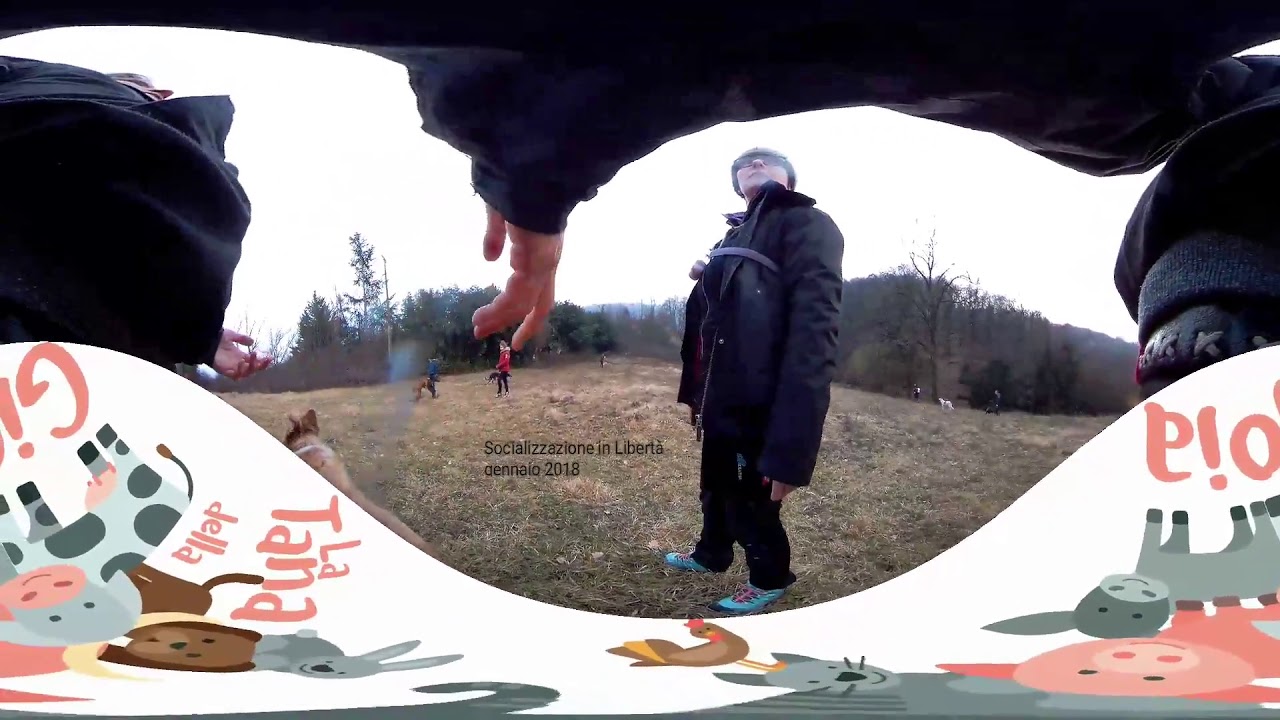The image captures an outdoor scene during the daytime, with lines distorted by the camera lens. At the center, there's a Caucasian man with a beanie cap and glasses, looking upwards to the left. He wears a black coat with a purple strap across his chest, black pants, and light blue sandals over red and white socks. His hands, mostly hidden by his coat, hang down near his knees. He stands on a field of mostly yellow, short grass with patches of green.

To his immediate right, there's a brown dog with pointed ears and a white collar. On the left side of the man, a hand extends out from a black piece of cloth, palm facing left and fingers straight down. Another dog appears on the far left of the image. Slightly behind the central figure, on the left, a person's head is visible, looking upwards and to the right, beneath which a hand with an open palm is seen.

In the background, a line of trees, including some pine and one dead tree on the right, frames the scene. Two additional people are seen behind the man, one in a red coat with black pants and another in a white jacket. The sky above them is white.

At the bottom of the image, there's a digital banner featuring colorful silhouettes of various animals such as rabbits, dogs, cows, chickens, cats, a donkey, and a pig, with light pink writing that includes "Latana Della" and possibly other text. The scene appears to have been captured in a wide-open field, suggesting a casual, social outdoor gathering.